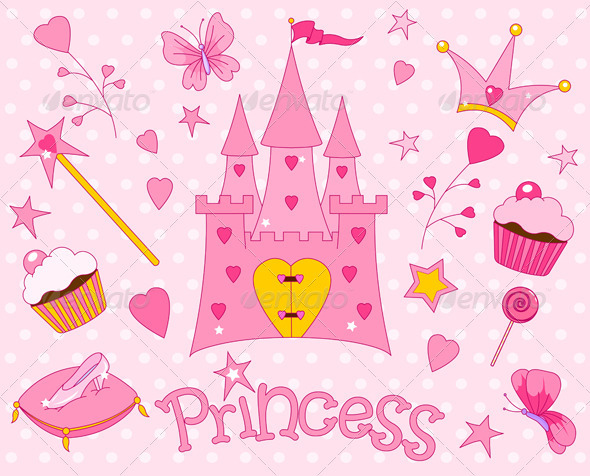The image is a cartoon stock photo featuring a highly stylized, whimsical design. The background exhibits a light pink color adorned with rows of evenly spaced white polka dots. At the bottom center of the image, the word "St. Princess" is inscribed in a playful Comic Sans font, with a star dotting the "i." 

Dominating the main center is a grand pink castle, embellished with hearts adorning all its towers and featuring a yellow door with a heart-shaped design. Encircling the castle, in a clockwise fashion, are various enchanting objects: a pink heel on a pillow, a crystal slipper on a pillow, a charming cupcake, a magic wand with a star encasing a heart, hearts on a branching element, and a delicate butterfly. Notably, the right side of the image displays additional items such as a crown with a heart motif, another cupcake, yellow and pink stars, a lollipop, and a second butterfly. The entire arrangement is festooned with pink and pink-accented hearts and stars, collectively enhancing the magical and royal theme depicted.

Subtly embedded into the background is a faded grid marking along with the faint text "Envato," indicating its origin as a stock photo. This adds a distinctive though subdued watermark, affirming its relevance for copyright or usage. Overall, the image exudes a whimsical, fairy tale-esque charm that is vividly detailed and visually captivating.